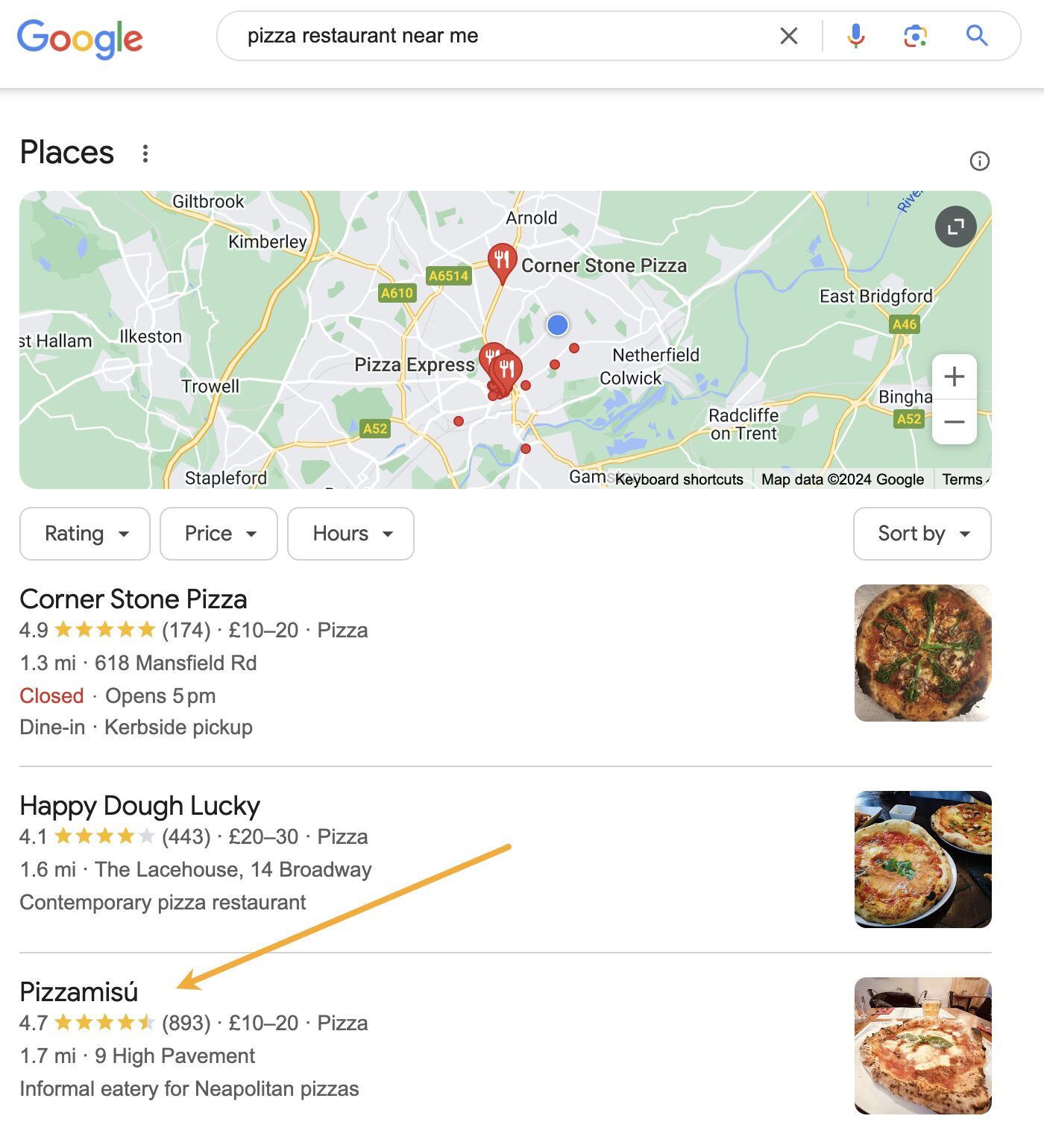This image showcases a Google search results page for "pizza restaurants near me". At the top left, the iconic Google logo is displayed. Adjacent to it is a search bar with the text "pizza restaurant near me" entered. Below this, there's a header labeled "Places" accompanied by a map featuring several marked locations, including Kimberly, Chowell, Stapleford, Radcliffe-on-Trent, and East Bridgeford. The map contains various red pins, each illustrated with a fork and knife symbol. Noteworthy pins include one labeled "Cornerstone Pizza" and another marked "Pizza Express". The bottom of the map cites "Map data ©2020 Google."

Underneath the map are three dropdown boxes with the texts "Rating," "Price," and "Hours" selected. The left column features search results starting with "Cornerstone Pizza," which is rated 4.9 stars, priced between £10 to £20, located 1.3 miles away at 618 Mansfield Road, currently closed but opening at 5 p.m., and offering dining and curbside pickup options. A photo of a pizza appears adjacent to this result.

The next listing is "Happy Dough Lucky," rated 4.1 stars, priced between £20 to £30, situated 1.6 miles away at The Lace House, 14 Broadway. It is described as a contemporary pizza restaurant, with a photo showing two pizzas next to it.

Following this, "Pizza Me Sue" is listed with a 4.7-star rating, pricing between £10 to £20, characterized as an informal eatery for Neapolitan pizzas. This entry is marked with a yellow arrow, and across from it is another pizza photograph.